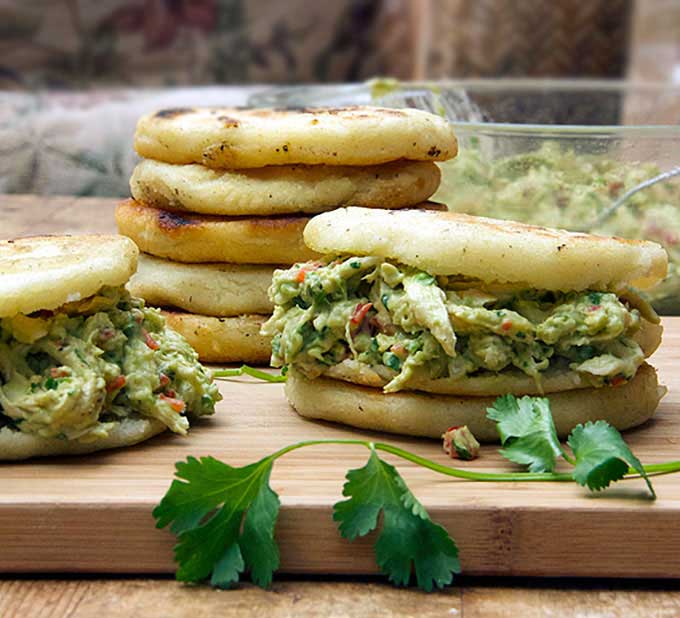The image showcases a well-staged, professional-looking photo of a delicious food arrangement set on a browned wooden table. At the forefront sits a wooden cutting board topped with two sandwiches made from flat, pita-like bread, resembling toaster biscuits. Each sandwich is filled with about an inch of a creamy, green mixture that likely includes avocado or guacamole, possibly mixed with peppers and chicken. In front of the sandwiches lies some fresh cilantro, adding a touch of green. Behind the sandwiches, centered between them, is a neat stack of five more of these pita-like breads. To the back left, there is a clear glass bowl containing more of the creamy green mixture, identified as guacamole, with a fork resting inside. This bowl also appears to have bits of red, probably from peppers, and hints of other ingredients. The background fades into a blur, revealing a material with floral patterns. The entire scene has a meticulously arranged, fresh, and appetizing appearance, indicative of a staged photo meant to highlight the enticing food setup.